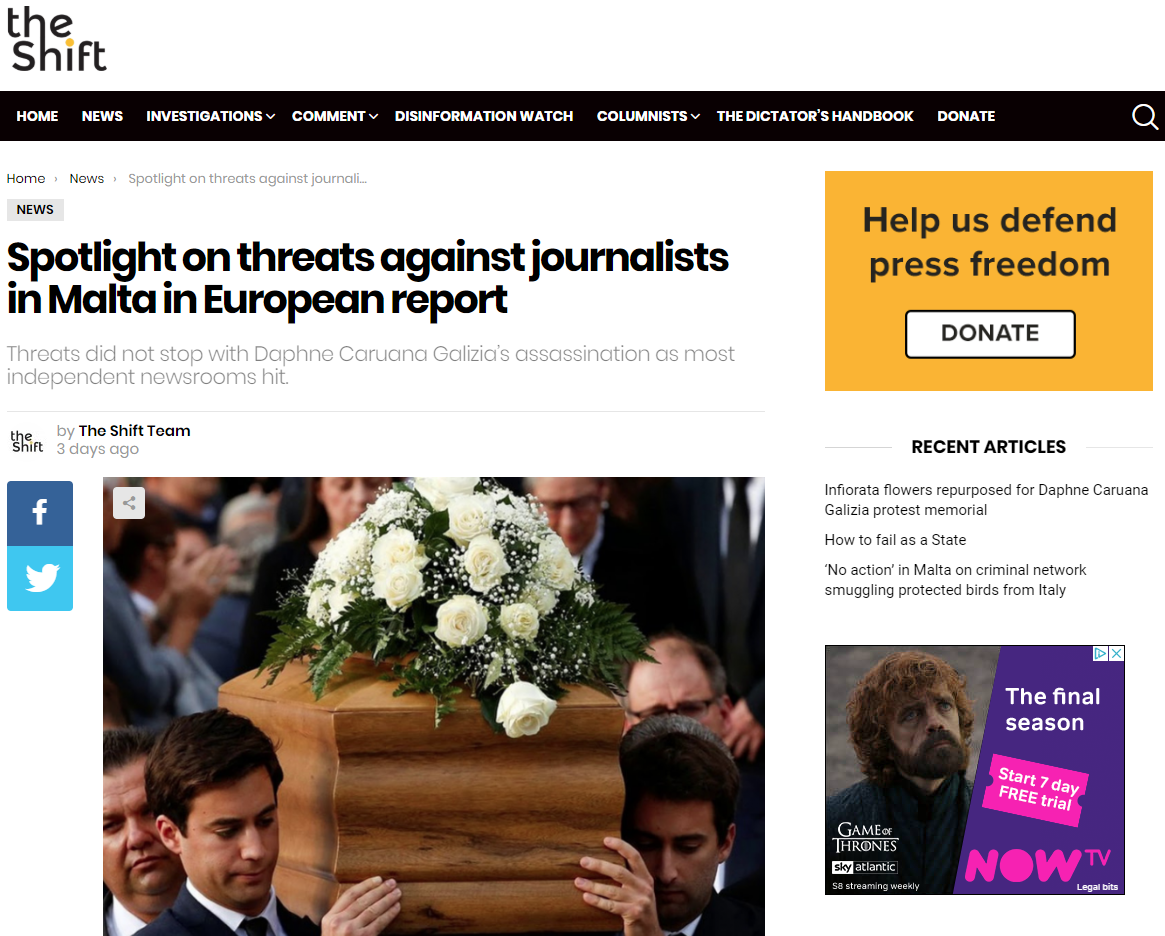This is a detailed screenshot of an article from "The Shift" website. At the top of the image, there's a black banner featuring white text displaying the various sections of the website. From left to right, the sections include: Home, News, Investigations, Comment, Disinformation Watch, Columnists, The Dictators' Handbook, and Donate. On the far right of the banner, there is a magnifying glass icon designated for searching.

Below the banner, the article's headline reads, "Spotlight on Threats Against Journalists in Malta in European Report". The subheading states, "Threats did not stop with Daphne Caruana Galizia's assassination; the most independent newsrooms hit." The article is credited to "The Shift Team" and was published three years ago.

In the lower portion of the image, there is a poignant photograph depicting two men who look strikingly similar, carrying a brown coffin adorned with white flowers through a crowd dressed in black.